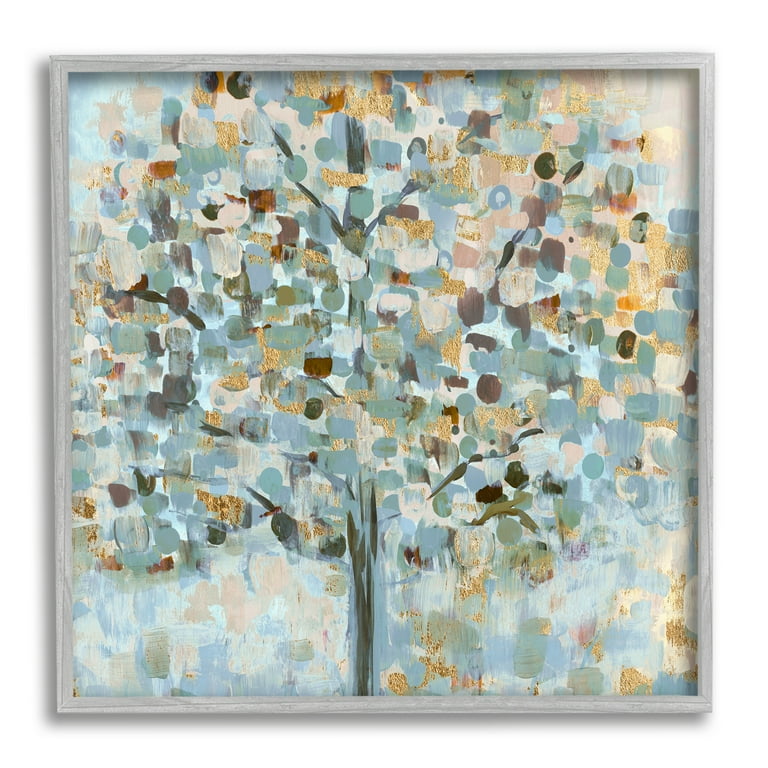This image captures a square painting framed in a gray wooden frame, reminiscent of a Monet with its dotwork style. It features a solitary tree with a narrow, greenish-brown trunk standing prominently in the center. The foliage is represented by an array of colorful dots, creating an impression of leaves. From afar, the dots coalesce to clearly depict the tree, while up close, they appear as individual dabs or smudges of paint. The leaves exhibit a spectrum of pastel tones, including white, gray, mustard, brown, light blue, creams, gold, and shades of green. The trunk and branches are defined with darker, straighter lines which contrast the more scattered and varied dots of the leaves. This meticulous arrangement of colors and shapes accentuates the abstract and modern art style of the painting. There is no text in the image, ensuring that the focus remains entirely on the detailed composition of the tree. The image is very clear, highlighting the intricate nature of the artwork.